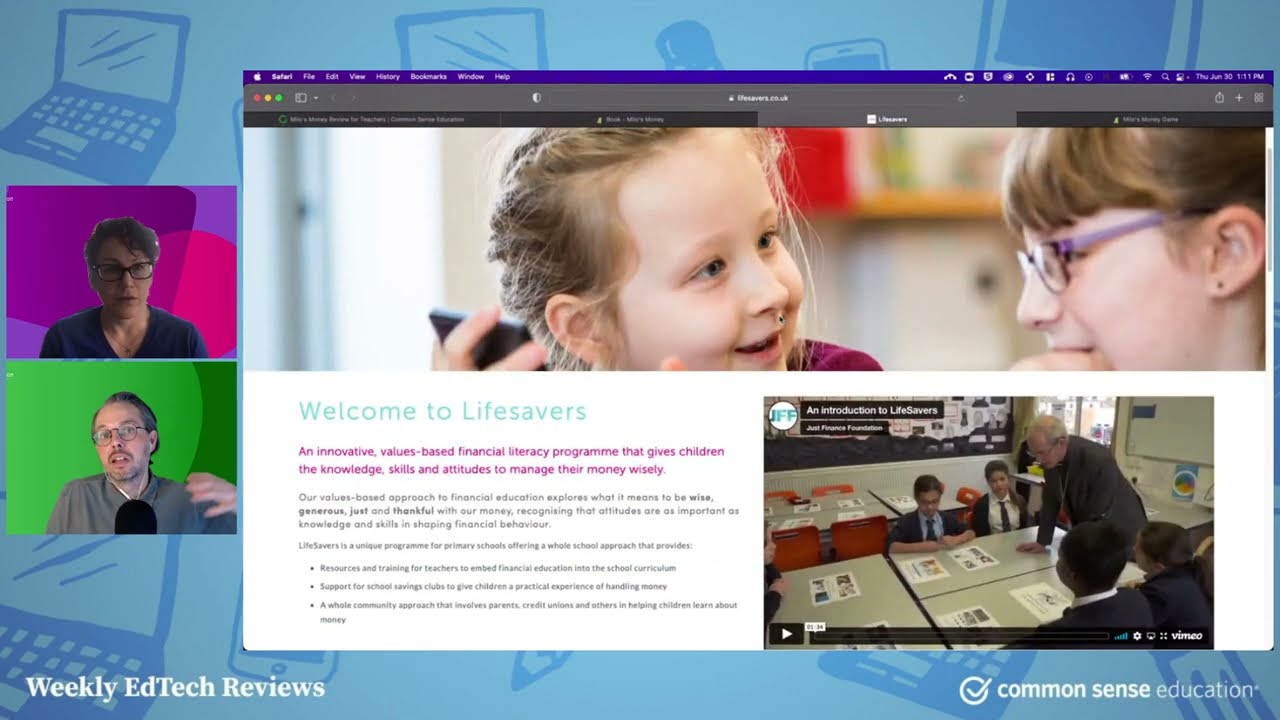The image illustrates a Zoom meeting featuring a website presentation prominently displayed at the center. The website, shown in a Safari browser with a blue background adorned with darker blue laptop and phone graphics, introduces the “Lifesavers” financial literacy program designed for children. The header showcases a banner image of two young girls, possibly in early elementary school, smiling at each other. The text reads, “Welcome to Lifesavers, an innovative values-based financial literacy program that gives children the knowledge, skills, and attitudes to manage their money wisely. Our values-based approach to financial education explores what it means to be wise, generous, just, and thankful with our money, recognizing that attitudes are as important as knowledge.” 

On the left side of the Zoom call, two webcam feeds are visible. The top one is a woman in a blue V-neck top with a necklace. She has short hair, black glasses, and a purple background with magenta shapes. Below her is a man with gray hair, wearing a button-up collared gray shirt and white earbuds. He also has glasses and is set against a dark and lime green background. Both individuals appear engaged in the video call, contributing to the presentation of the Lifesavers program. The bottom of the web page features affiliations with "Weekly EdTech Reviews" on the left and "Common Sense Education" on the right.